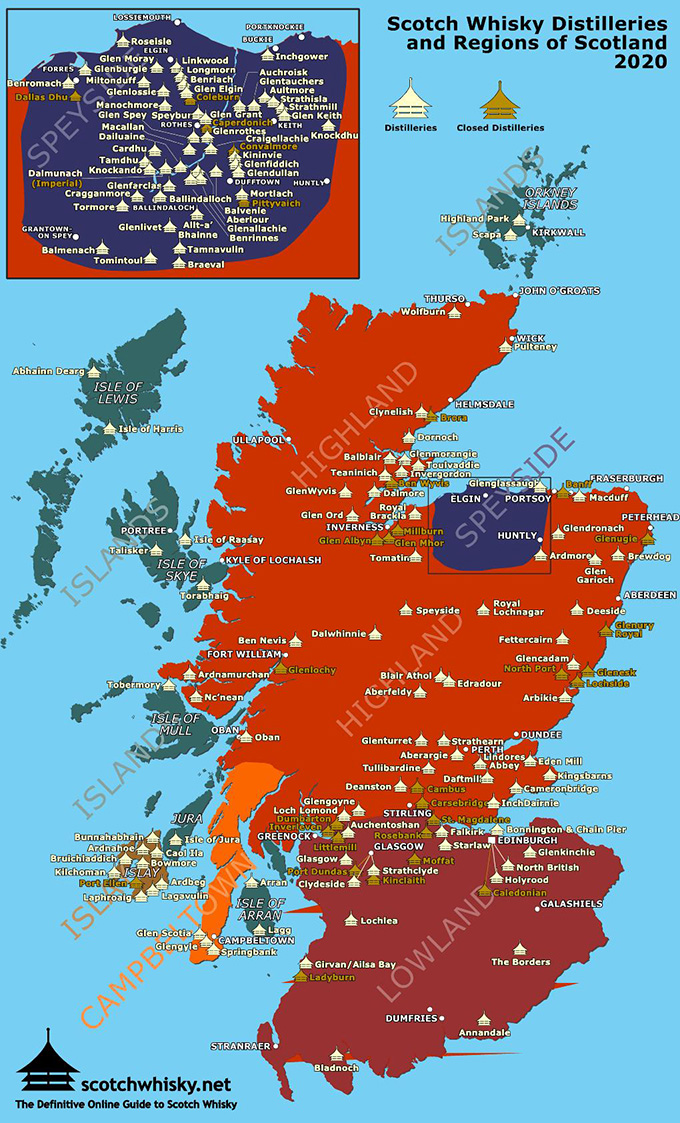The image is a detailed map titled "Scotch Whisky Distilleries and Regions of Scotland 2020." The map predominantly shows Scotland, divided into various whisky-producing regions. The Highland region, marked in a dark red, is the largest section. Below it, the Lowland region is indicated in maroon. To the left is Campbeltown, highlighted in orange. Islands surround these main areas, including the Isle of Lewis, Isle of Skye, Isle of Mull, and Orkney Islands, drawn in a teal color. The background of the map is light blue, representing the ocean. 

The top left corner features a close-up section, with detailed locations of several distilleries. White symbols denote open distilleries, such as Dab Munch, Braviol, Mildentuff, Rosell, Linkwood, and Longmore. Beige-gold symbols indicate closed distilleries like Colborne, Conovermore, and Pityvac. The legend at the top identifies the symbols and regions. At the bottom, black text reads "scotchwhisky.net, the definitive online guide to scotch whisky."